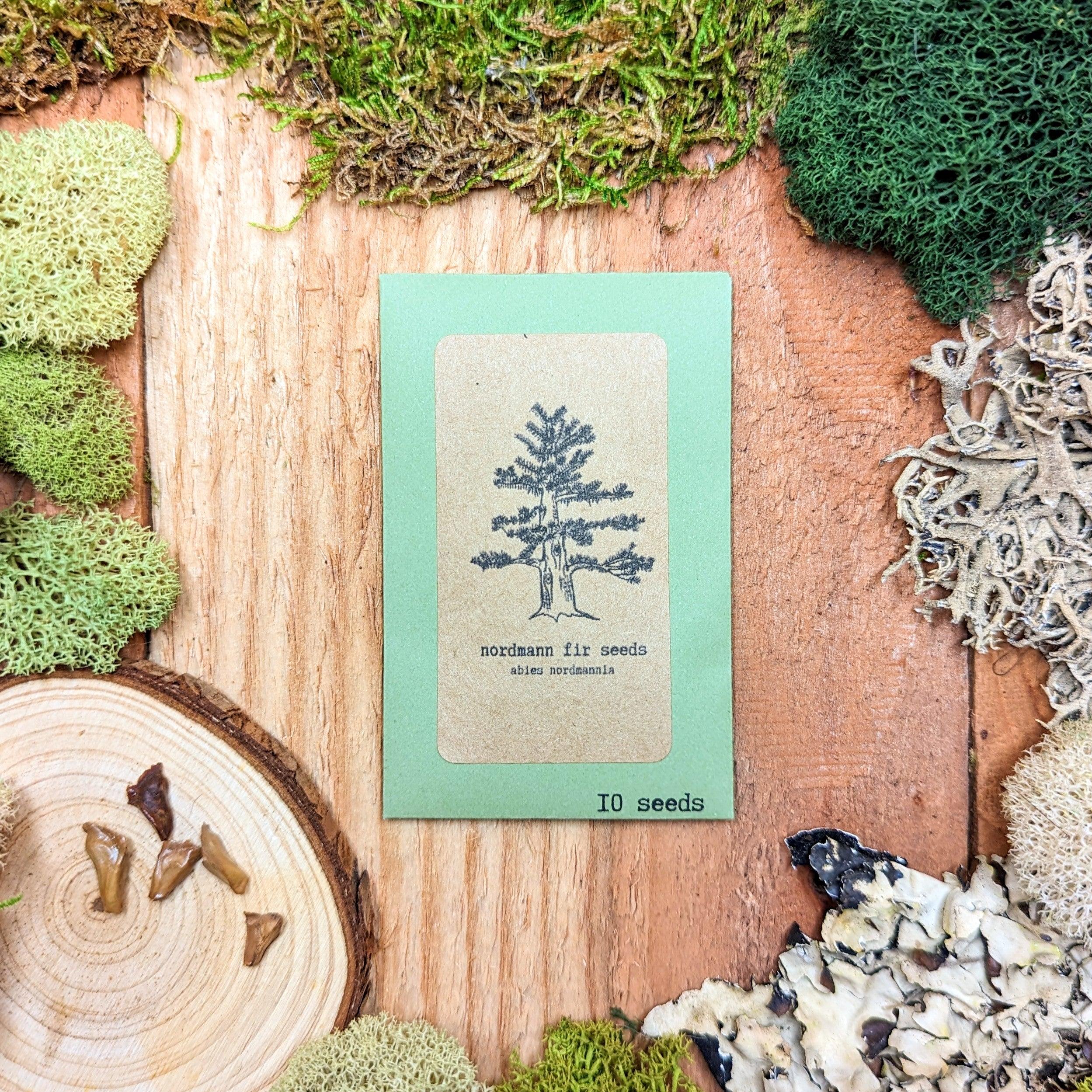In the center of the photograph is an aqua-colored packet of seeds, with an off-white label bearing an illustration of a fir tree in blue ink and the words "Nordman Fir Seeds, Abies nordmanniana" beneath it. The packet promises seeds that can grow into large Nordmann fir trees and contains ten seeds. The packet is artfully placed on a wooden table composed of planks, surrounded by various types of foliage. The table features a circular tree stump in the bottom left corner and is bordered by an assortment of green and white vegetation, including grasses and seaweed-like plants. There are also shiny rocks or artifacts among the foliage, contributing to the forest-like, natural ambiance of the photograph.